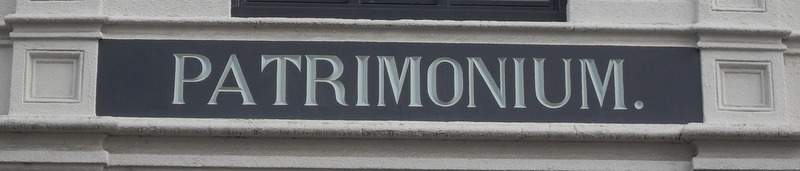This photograph captures a close-up of an ornate sign on the facade of an older, likely neoclassical stone building, suggesting an age of over a hundred years. The building is constructed from white stone with a textured appearance, resembling classic Greek architecture, potentially featuring columns, although they are not visible in this image. The focus of the photograph is on the sign itself, which is centrally placed against a black background strip. The sign displays the word "PATRIMONIUM." in all capital letters. The characters are embossed and appear to be painted in a light greenish or grayish hue. The sign is flanked on each side by large carved squares that are integrated into the building’s stonework, bordered by grooves, giving it a framed look. The sign is set above a decorative strip that serves as a ledge, potentially over a doorway or entrance, and runs between two levels of the edifice. The craftsmanship of the building and the sign reflect a level of heritage and historical significance, adding to the overall grandeur of this architectural element.